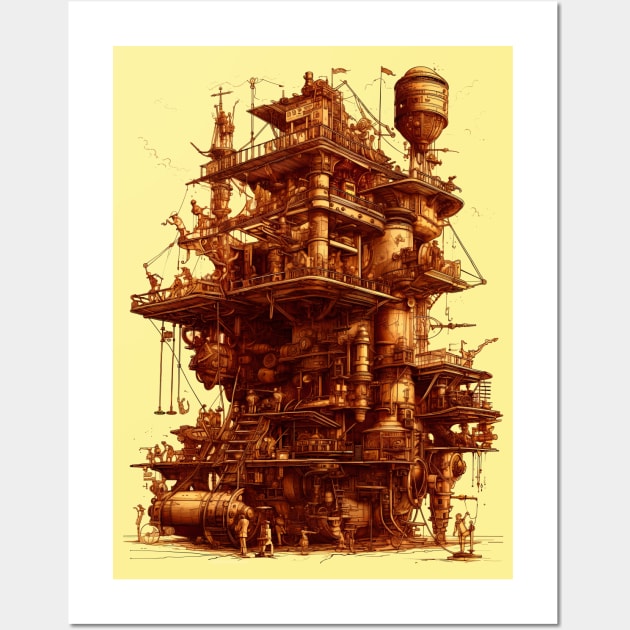This detailed sketch, primarily in black and white with a yellow and orange overlay, depicts a complex, multi-story, steampunk-inspired structure resembling a hybrid between an industrial oil rig, a ship, and an apartment building. The illustration showcases a towering edifice with numerous platforms and railings, each layer interconnected with various pipes, conduits, ladders, and cylindrical components. At the pinnacle of the structure sits a prominent water tower, with multiple flags fluttering, indicating an outdoor setting. Intricate details such as gears, pulleys, cables, banisters, and ropes adorn the frame, contributing to its half-machine, half-dwelling appearance. The design suggests a bustling environment, possibly inhabited or operated by people, although individual figures are subtle or not distinctly visible. The overall aesthetic, with its sepia-toned ink drawing or painting style, evokes a steam-powered, futuristic allure, set against a plain background, making it seem like a highly detailed poster illustration.